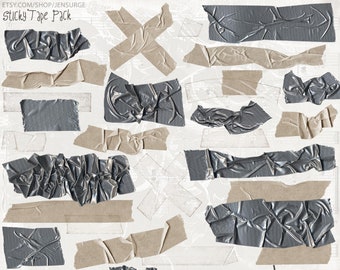The image, titled "Sticky Tape Pack," prominently features an assortment of crinkled and layered tapes on a light white or off-white background, which might be a piece of paper or cardboard. In the top left corner, the text "STICKY TAPE PACK" is visible along with a small, partially readable website, possibly etsy.com/shop/jensurge. The collage comprises various types of tape including gray, brown, white, beige, and some clear, with each piece exhibiting a unique texture — some are smooth, others are twisted or torn. The tapes are arranged in different orientations, with several pieces laid horizontally, a few forming an X pattern, and others simply overlapping, creating an intricate and tactile visual presentation. The majority of the shapes are rectangular, varying in size, emphasizing the chaotic yet structured nature of the displayed tape assortment.